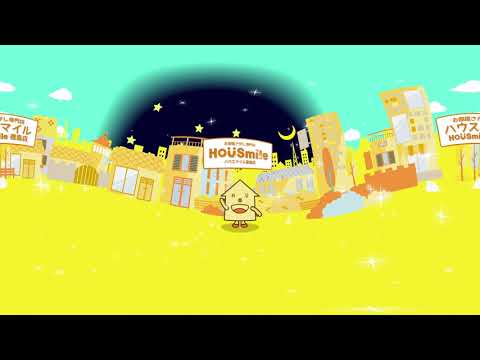The image is a cartoonish, animated scene featuring a human-like, yellow house standing on a vibrant, neon yellow hilly ground. The house has a rudimentary, happy face with windows as eyes and a window as its nose. Its arms stretch diagonally towards the top left corner. The background behind this smiley house depicts a village with a row of buildings and stores adorned with Japanese characters on white rectangular signs in orange font.

Above the anthropomorphic house is a banner reading "HOU Smile," with the letter "U" designed as a smiley face. The sky displays an unusual gradient, transitioning from bright teal to a patch of night sky featuring a yellow crescent moon, yellow stars, and some twinkling white stars. The surroundings are primarily various shades of yellow, with the buildings carrying yellowish-orange hues and blue and orange accents. The image is horizontally letterboxed, giving it a cinematic feel, suggesting it might be a scene from a television show or an ad.